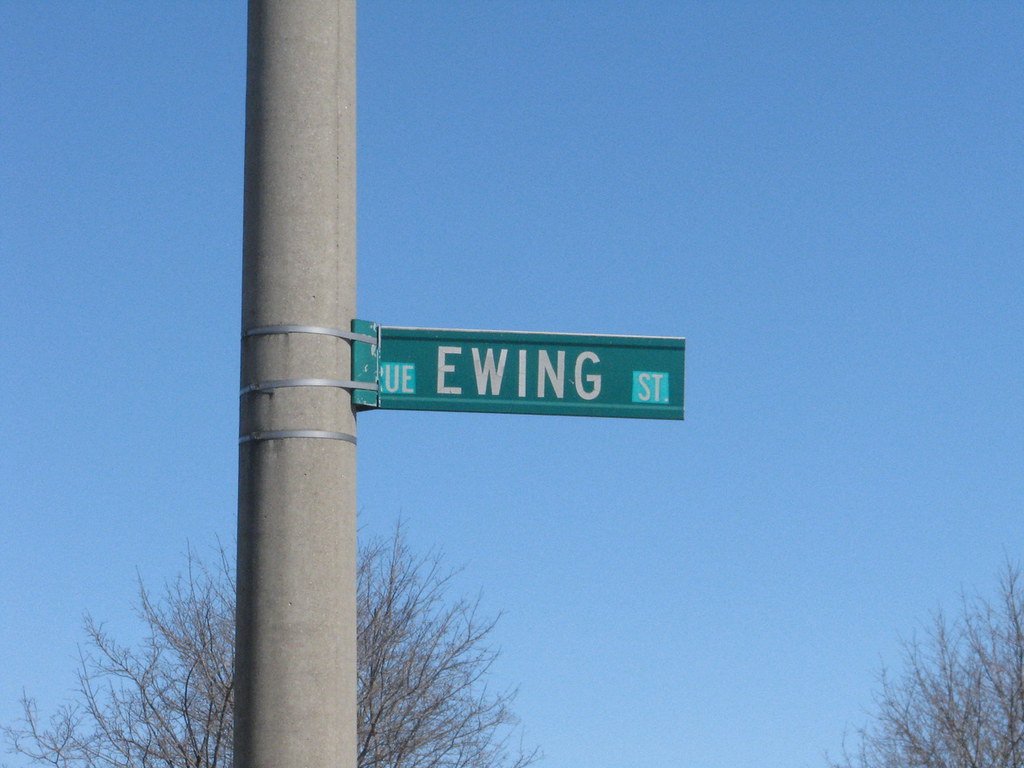The photograph captures an upward view of a green rectangular street sign reading "Ewing Street" in white reflective capital letters. The sign is fastened to a large, cylindrical metal pole with three silver bands. The pole and sign are framed against a vivid, cloudless blue sky that subtly transitions from a medium blue at the top to a slightly lighter shade near the bottom. Complementing the scene, bare-branched trees, indicative of winter, are visible at the image's lower corners, their spiky, leafless branches extending upwards. The overall image emphasizes a contrast between the serene sky and the stark, wintery trees, with the street sign prominently centered.